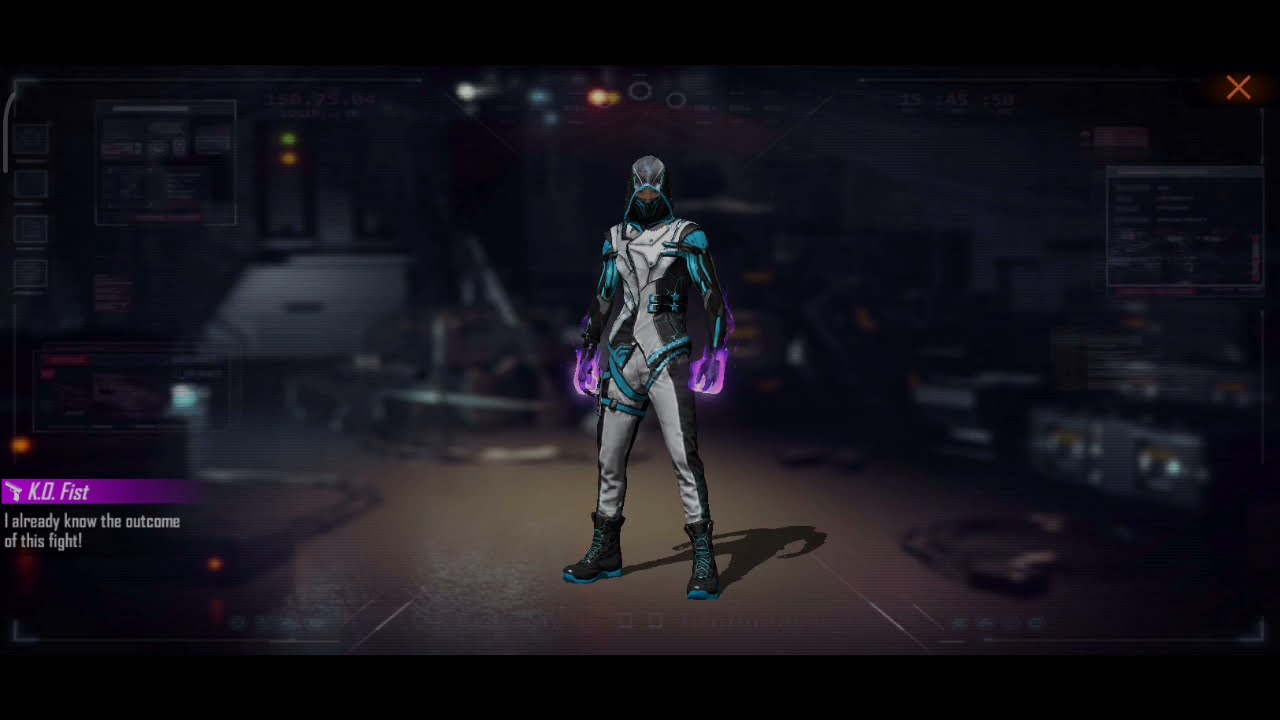The image is a rectangular screenshot from a video game, featuring a central character in a dimly-lit, factory-like environment with a blurred background of mechanical equipment. The floor is shiny and brown. Dominating the image is a character standing proudly in the center, wearing a light gray bodysuit with dark gray outlines and turquoise accents. His look is completed with a hood and a black mask featuring turquoise details that cover the lower part of his face. His hands are dramatically encased in glowing purple flames, suggesting imminent action. On the left side of the image, a purple banner with white text reads "KO FIST," followed by, "I already know the outcome of this fight," hinting at a fighting game scenario. In the upper right corner of the screenshot, there is a red "X" icon, typically used to close the screen. The overall atmosphere is tense, as if the character is poised for battle or a critical moment within the game.